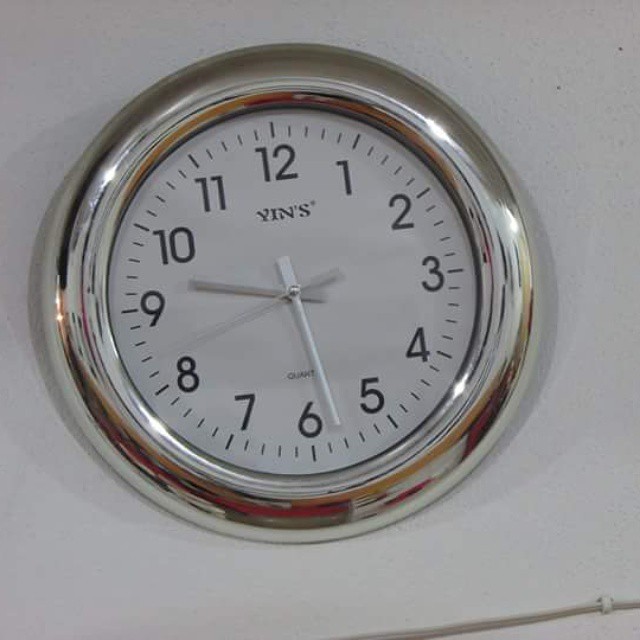A large, chrome wall clock with a thick, rounded frame dominates the scene. The frame's highly reflective surface catches the room's lighting and various colored objects, creating a dynamic interplay of reflections. The clock displays the time as 9:28, with the second hand precisely pointing at the 42-second mark. The timepiece is branded by "Vin's," with the name elegantly inscribed near the top. The word "Quartz" appears at the bottom of the clock face, signifying its mechanism. The face itself is a pristine white, featuring bold, black Arabic numerals ranging from 1 to 12. The clock is mounted on a white wall, where a neatly tacked white wire is visible just below it, adding a subtle touch of functionality to the otherwise classic aesthetic.